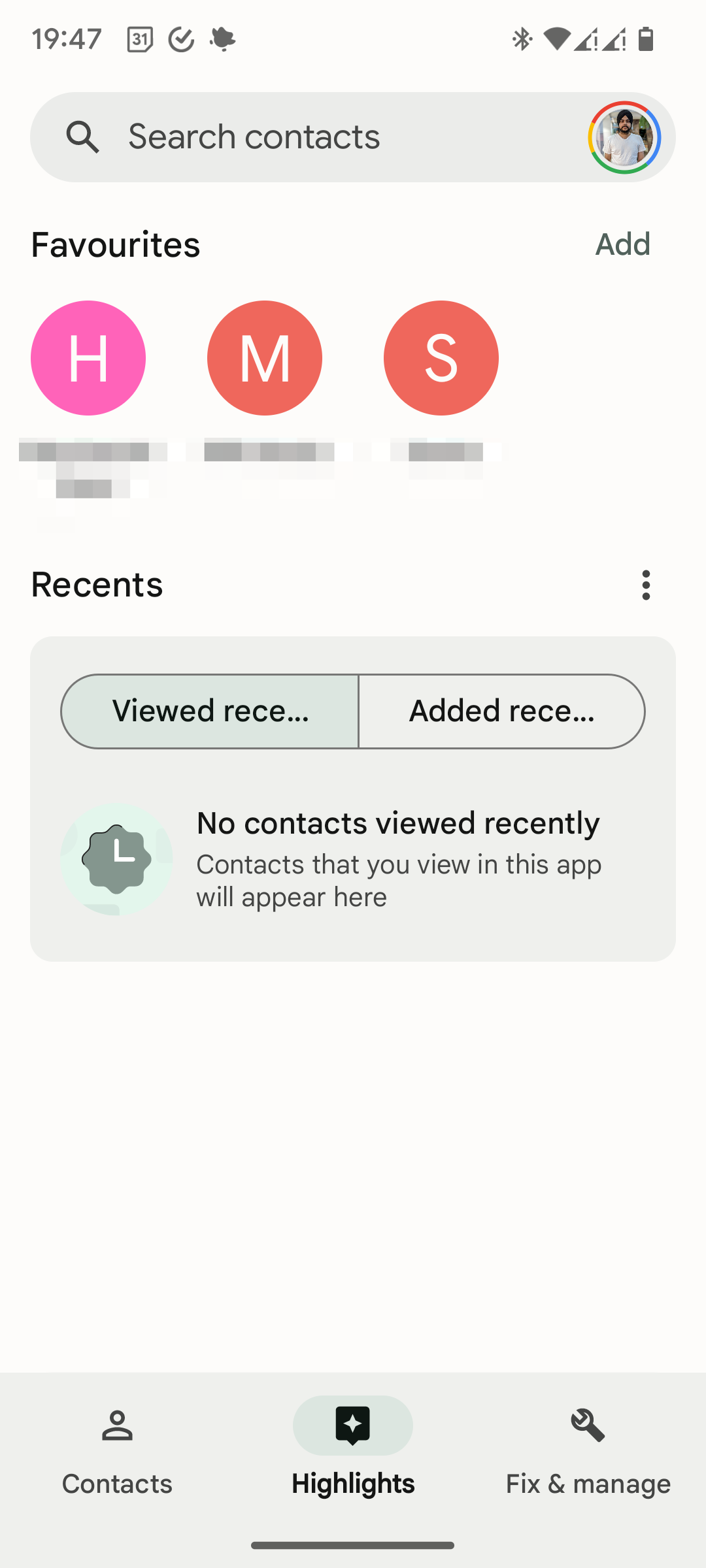The image features a user interface layout against a light purple background. At the top, the year "1947" and the date "31st" on a calendar are prominently displayed next to a circle with a checkmark. Below, a search box is positioned alongside a colorful circle - comprising red, yellow, blue, and green segments - containing a person's picture. Nearby, the word "Favorites" is inscribed with an option to "Add" on the far right.

To the right, three circles are visible: a pink one with an "H," a red one with an "M," and another red one with an "S." The content directly below these circles is obscured. Underneath, the heading "Recents" appears above a blue box with two buttons labeled "Viewed Recently" and "Added Recently." A small clock icon is situated to the left of this section.

Additionally, a message stating "No contacts viewed recently. Contacts that you view in this app will appear here" is visible within the blue box. At the bottom, another blue menu bar features options for "Contacts," "Highlights," "Fix and Manage," separated by a black line. This interface organizes features such as favorites and recent contacts, allowing users to view and manage their contact interactions effectively.